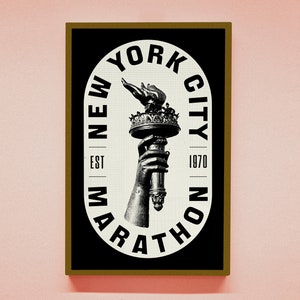This image is a detailed digital creation resembling a framed poster for the New York City Marathon. It has a distinctive design with a black rectangular backdrop bordered by a brown frame. The background behind the frame transitions from a dark pink or maroon at the bottom to a light pink or carnation around the rest of the frame, suggesting a shadow effect.

At the center of the black rectangle is a large, white oval that is taller than it is wide, resembling a stretched pill shape. Encircling the edge of this oval, the text "New York City" is inscribed at the top while "Marathon" is written along the bottom. On the left side of the oval, the abbreviation "EST." is placed, indicating the year of establishment, which is marked as "1970" on the right side.

Within this white oval, there is a black and white sketch depicting the hand of the Statue of Liberty holding up her iconic torch. The entire composition has a monochromatic palette with the text and drawing in black, adding a classic touch to the modern design.